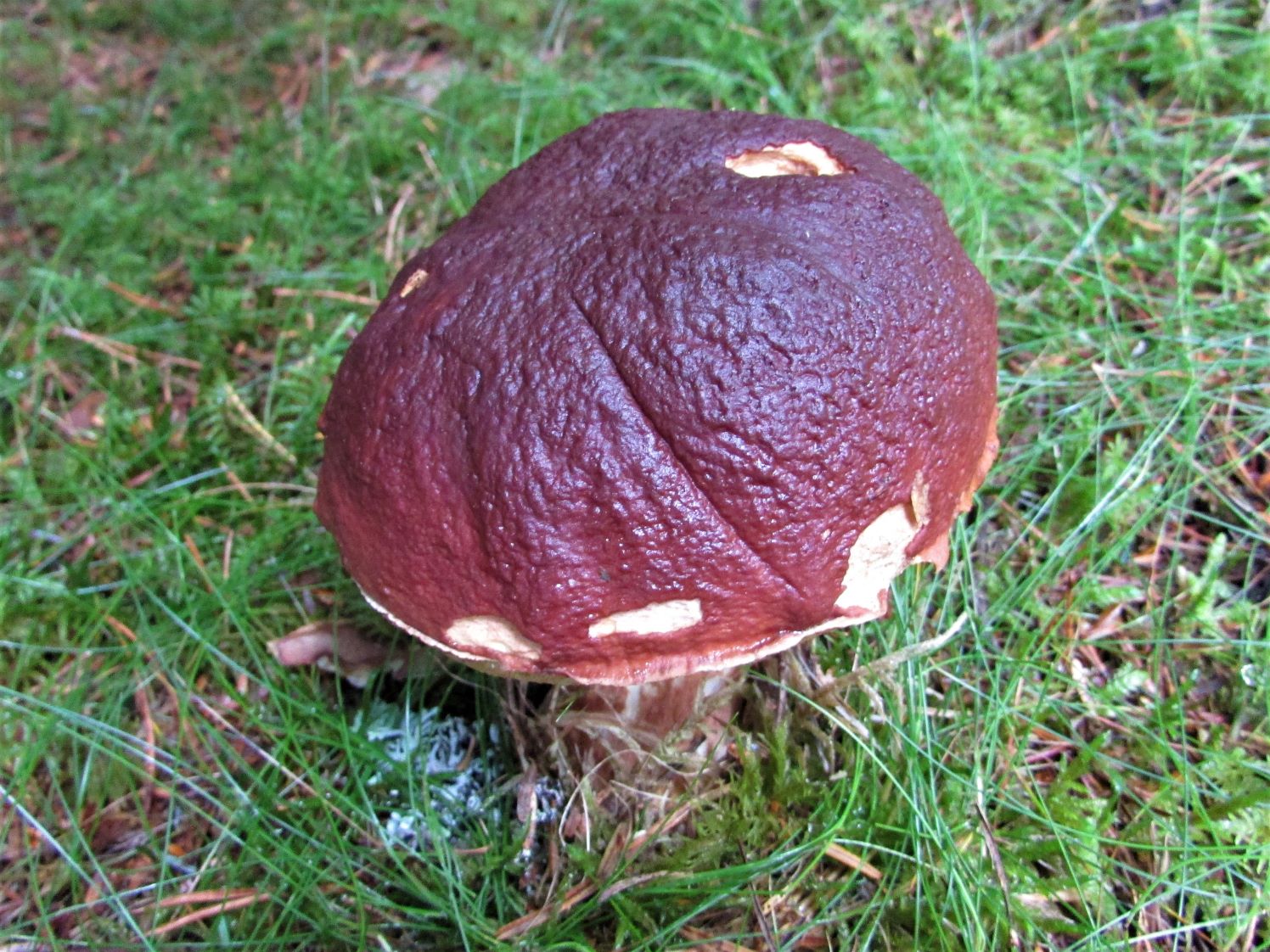This detailed close-up photograph captures a striking image primarily focused on a single mushroom. The mushroom, standing about 3 to 4 inches tall, is set against a background of sparse, short grass that barely reaches its height. Its cap is predominantly a dark brown, almost burnt in appearance, with multiple spots where the outer layer has flaked off, revealing a beige to white interior. This gives the mushroom a somewhat wrinkly, bumpy texture reminiscent of a loaf of bread. The composition primarily shows the top of the mushroom, but a few white spots are evident underneath the cap, and glimpses of the stem are visible as it emerges from the ground. The image is devoid of any distinct features in both the background and foreground, ensuring that the viewer's attention remains solely on the intriguing textures and colors of the mushroom.